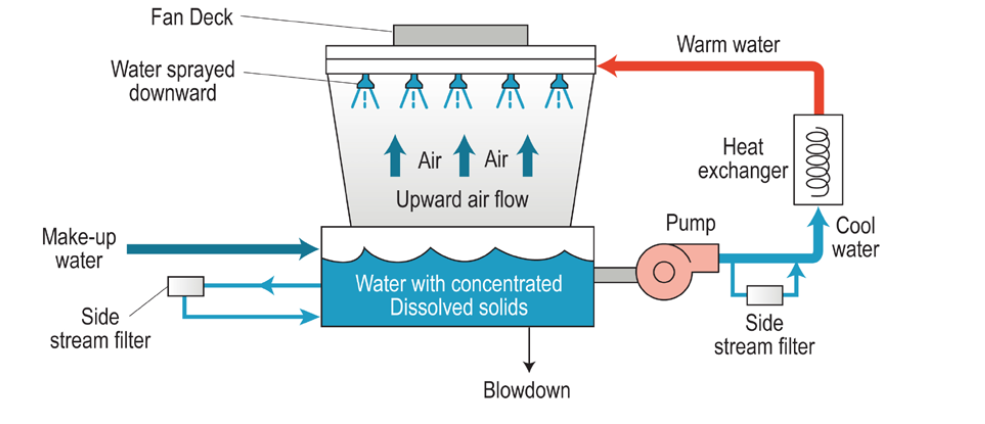The image depicts an intricate flow diagram of a mechanical cooling system. At the center, there's a large black-bordered rectangle labeled "Water with Concentrated Dissolved Solids." Below this rectangle, an arrow marked "Blowdown" points downward. Above the rectangle sits a parallelogram-shaped device with five blue showerheads, spraying water downwards onto three upward-facing arrows labeled "Air." Between the arrows, the term "Upward Airflow" is mentioned.

At the top of this configuration is a smaller rectangle titled "Fan Deck." On the left side of the diagram, a blue line labeled "Makeup Water" leads towards a square marked "Sidestream Filter," from which an arrow points to the right towards a pump. This pump is connected via another line leading to the right and then upward towards a coil-shaped drawing labeled "Heat Exchanger." A red line emanates from the heat exchanger, marked "Warm Water," and directs to the left side of the system, showing the heating process.

The illustration employs blue coloring to indicate the path of water and red for the warm water path, providing a clear visual distinction between the two. Overall, it seems to be a detailed instructional layout of a cooling or water treatment system, highlighting the flow of water and air through various components like pumps, filters, and heat exchangers, all topped with a fan deck for managing airflow.